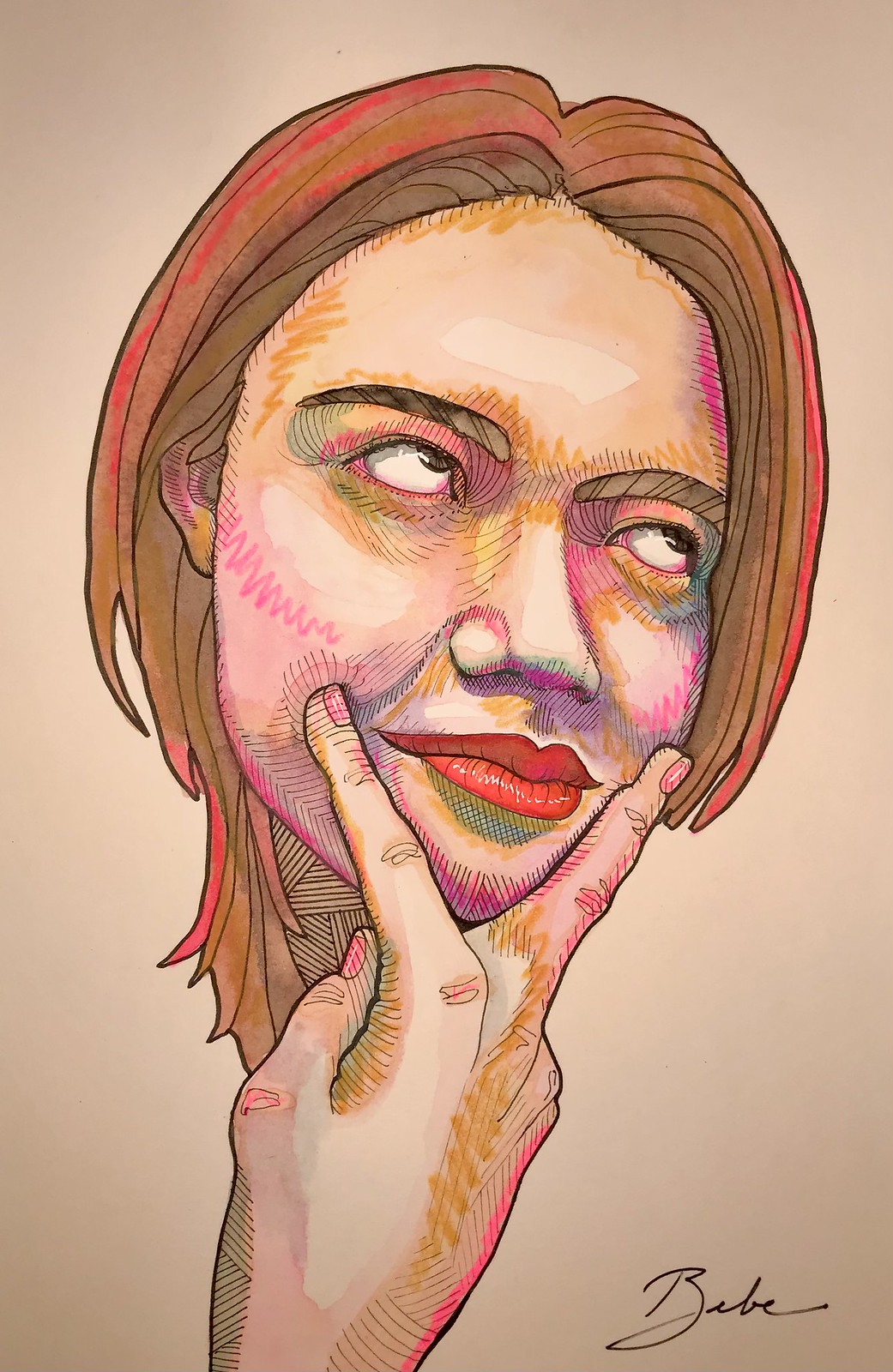This drawing, potentially created electronically or with traditional media like markers and colored pencils, features an intricate, stylized portrait of a woman with a straight face, reminiscent of Angelina Jolie. The woman has short brown hair with pink highlights, parted in the center and draping down to her neck, which is not visibly attached to her head. Her expressive, full eyebrows frame her eyes, which are gazing upwards to the upper right, revealing mostly the whites and hints of gray. 

The detailed shading on her face incorporates unexpected yet harmonious hues of yellow, pink, blue, and green, enhancing the natural contours and features. She wears striking red lipstick on her full lips. Her right hand is prominently positioned near her face, with the index and middle fingers spread apart to frame her chin and lips. The fingers, adorned with pink nail polish, exhibit subtle pink and yellow shading, adding depth to the hand's depiction. 

The background is a neutral beige tone, bringing focus to the vivid details of the portrait. The drawing is signed in cursive "Bebe" in the lower right corner.